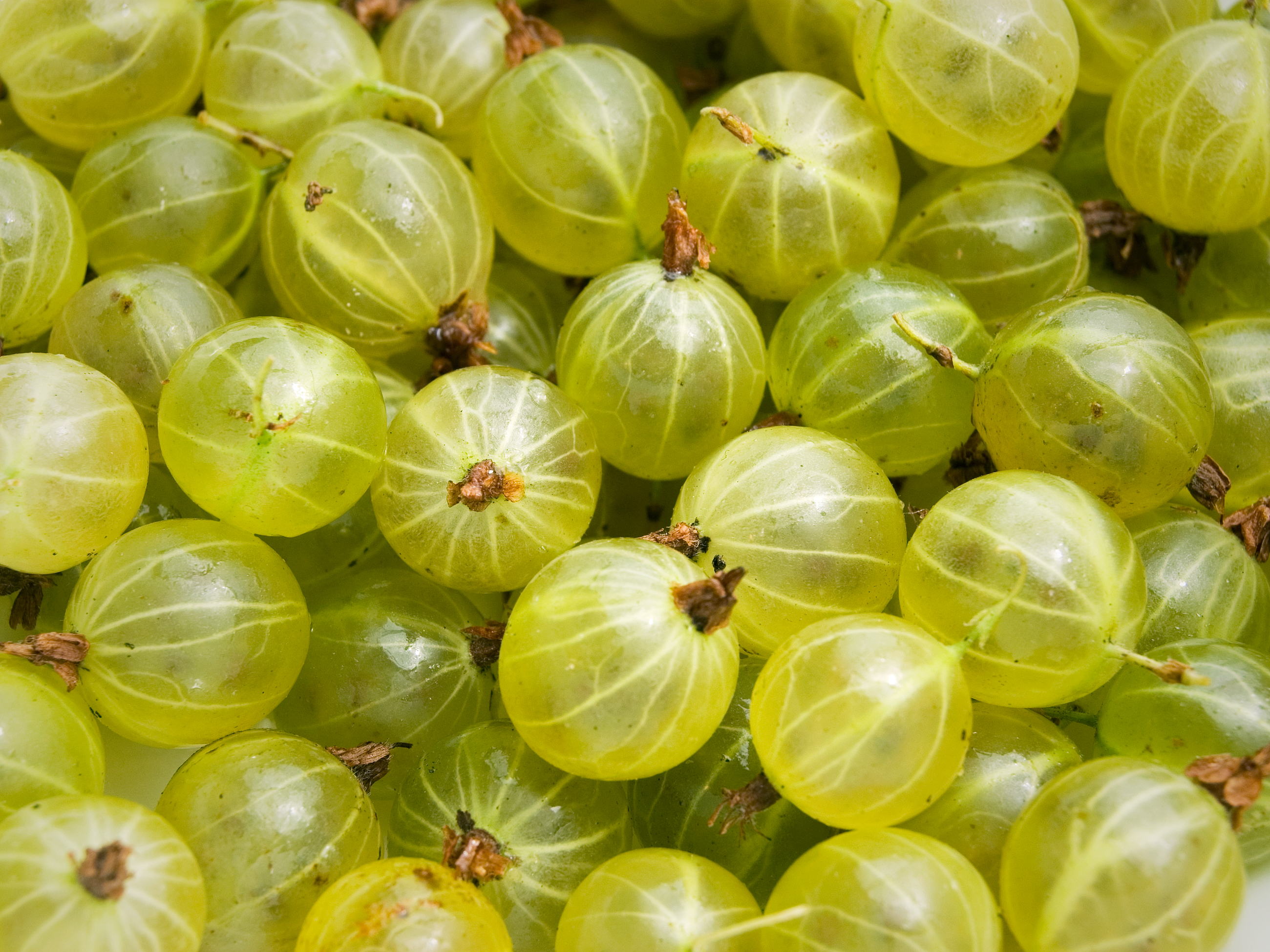The image depicts a close-up, highly detailed photograph of what appears to be green grapes, although they exhibit some unique characteristics that make them somewhat different from typical grapes. The grapes are small, orb-shaped, and have a translucent quality, allowing a subtle glimpse into their interiors. They are covered in light, vein-like patterns running through their surfaces, which are described as white veins. A cluster of these green grapes is piled together, with many of them sporting short brown or green stems extending from their tips. The grapes appear wet, giving them a juicy texture, and there are occasional specks of dirt, possibly from the stems. The background is somewhat unclear due to the tight zoom on the grapes, but hints of white suggest they might be placed on a plate or in a bowl. Overall, the image offers an intricate view of these unique, grape-like fruits.